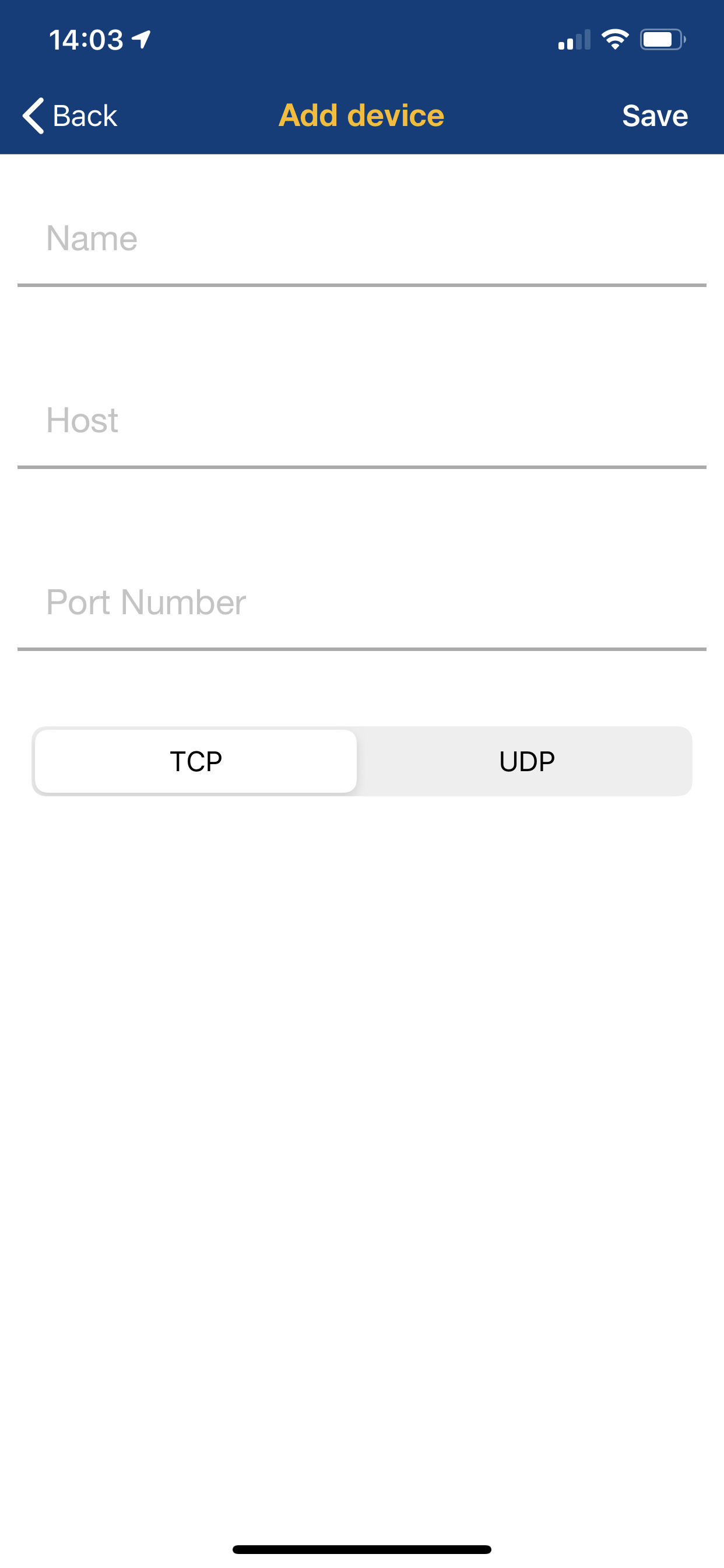The screenshot displays a phone screen with the top part featuring a navy blue background. In the upper left corner, the time is shown in white as "14:03," accompanied by a rightward-pointing arrow. Adjacent to this, on the upper right, there are two out of four white bars indicating cellular reception strength, suggesting moderate signal quality. The Wi-Fi signal, represented by a white icon, indicates strong connectivity. The battery icon, predominantly white and around 80% full, is also visible.

Beneath this section, towards the left, there's an arrow pointing left with the label "Back" next to it, each word commencing with a capital letter. The center of the screen features the word "Device" in yellow with a capital "A." To the right, the word "Save" is displayed with a capital "S." The background transitions to white below these elements.

In this white section, several fields are listed in gray text, each starting with a capital letter. There are labels such as "Name," "Host," and "Port Number," each followed by a thin gray line that spans the width of the screen. Underneath the "Port Number" section, there's a gray rectangle with "UDB" written in black, capital letters on the right side. Within this gray rectangle, a smaller white rectangle contains the label "TCB" in black, capital letters.

The overall layout suggests a configuration or settings page likely related to network or connectivity settings on a device.